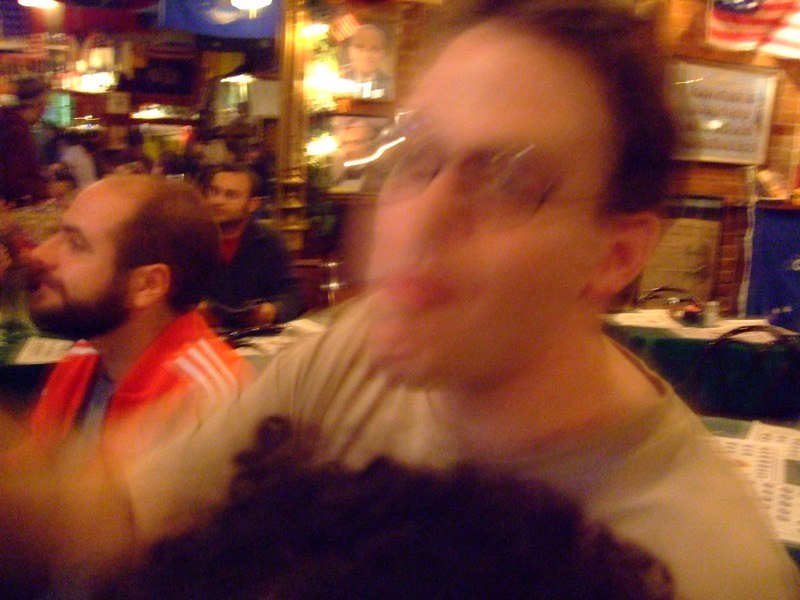In this slightly out-of-focus image captured inside a bustling restaurant or bar, a man takes center stage on the right side of the frame. He is dressed in a tan shirt and wears glasses. Notable details include his receding brown hair and pursed lips. In the foreground, the top of another person’s head with curly brown hair is visible. To the left of the central figure, another man appears facing away to the left. He sports a bearded mustache and also has receding brown hair. He is dressed in an orange athletic jacket featuring three stripes on the shoulders, layered over a gray T-shirt. The background reveals a lively setting with numerous patrons on the left side, and the right-hand side adorned with various signs on the wall. A table with a blue tablecloth is conspicuously set in the center-right, adding to the scene's warm, social atmosphere.